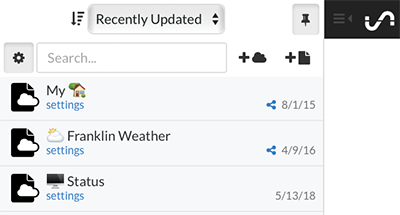The image is a horizontally oriented rectangular screenshot showcasing a segment of a phone's settings menu. The background is predominantly white, with three options displayed on gray backgrounds. In the upper right corner, there is a small, short black rectangle. 

Towards the right-hand side, there is an icon resembling a sideways 'S' with a horizontal line through it. Adjacent to this icon is a three-line menu, accompanied by a left-pointing triangle positioned to its right. On the left side of the screen, a drop-down menu button labeled "Recently Updated" in black text appears, followed by an image of cascading lines with a downward-pointing arrow. To the right of this, there is a thumbtack icon button.

Beneath this row, the next line features a settings icon (depicted as a gear) situated next to a search bar. Following the search bar are a plus sign, a cloud icon, another plus sign, and a file icon. 

Below these buttons, there are three options, each symbolized by a file icon with a cloud overlay. The first option reads "My Home Settings," accompanied by a home icon and a date of "8-1-15." The second option is labeled "Franklin Weather Settings," featuring an icon of a cloud with the sun peeking behind it and a date of "4-9-16." The third option shows a computer monitor icon with the word "Status" and "Settings" beneath it, along with a date of "5-13-18."